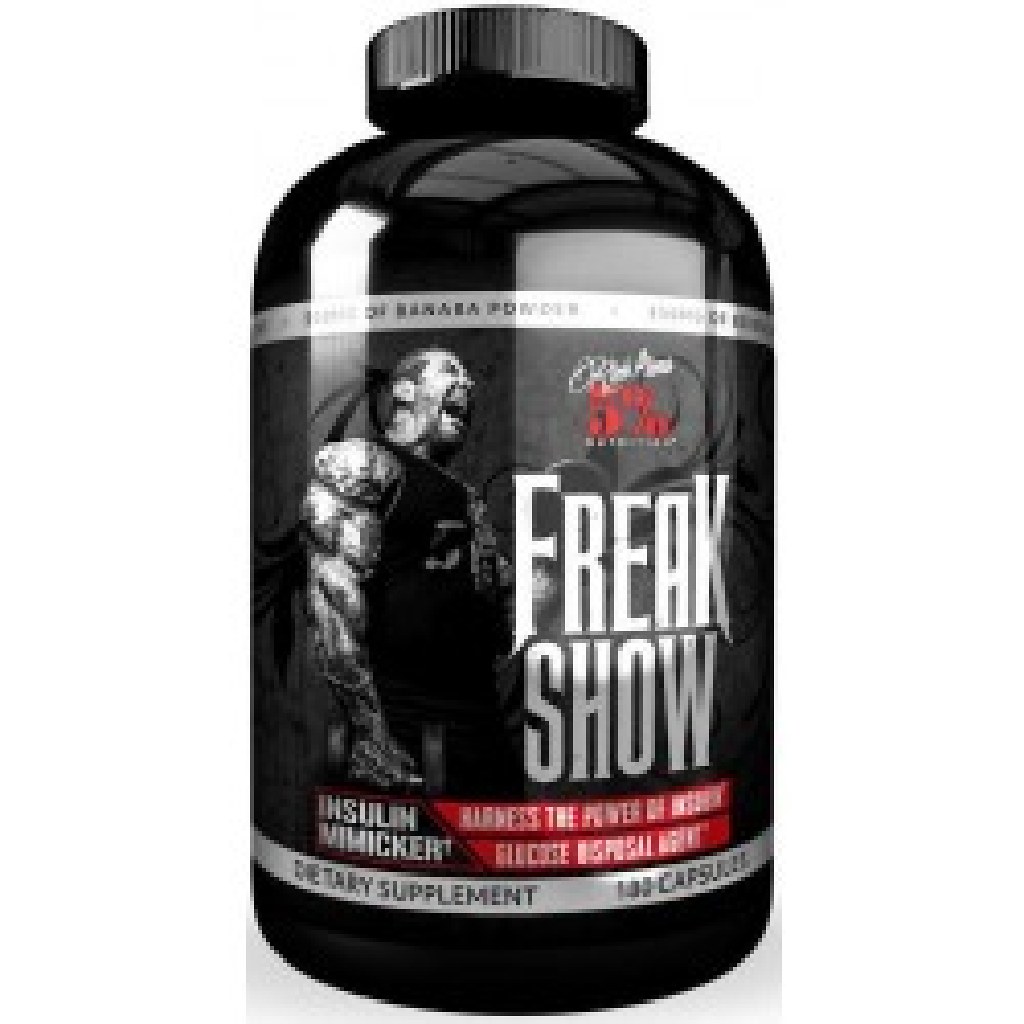The image depicts a black, cylindrical bottle of a dietary supplement named "Freak Show." The bottle, made of shiny black plastic, features a matching black lid. Despite the slight blurriness of the photo, some details remain discernible. The primary label includes bold white lettering prominently stating "Freak Show" with the phrase "insulin mimicker" written beneath it, indicating the supplement's function in insulin regulation. 

A striking image of a muscular, intensely screaming man wearing a black shirt graces the label; he appears to be flexing his muscles or holding barbells. The label also includes a silver, white, and black design with red accents, though some of the text is hard to read. To the right of the main label area, there is a red background with white text that mentions "glucose." The bottom part of the label notes that the bottle contains dietary supplements, with the exact count of capsules being over a hundred but not clearly visible due to the blurriness.